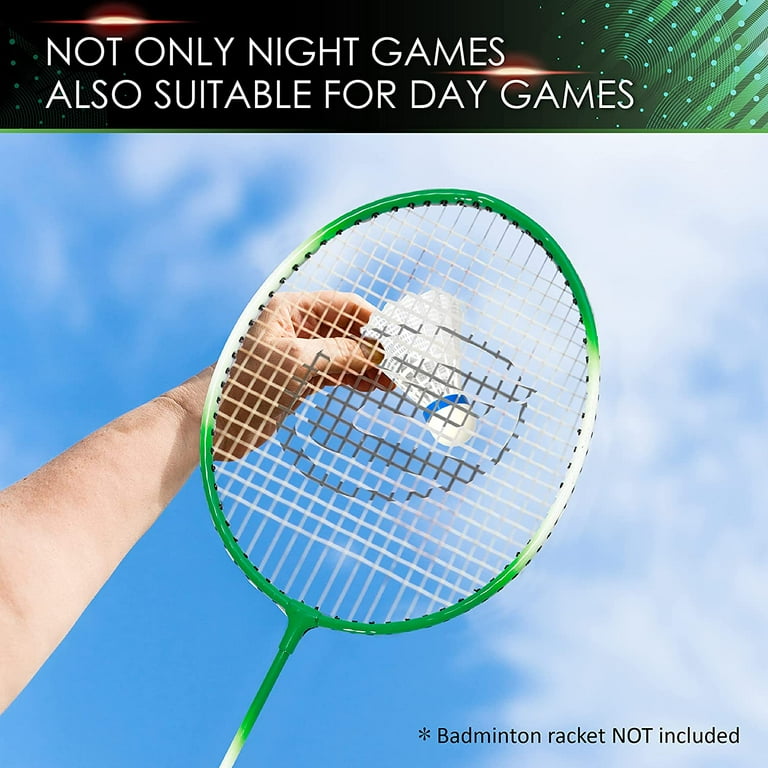The photograph captures a vivid outdoor scene with a striking, bright blue sky adorned by a few soft, white clouds. Dominating the composition is a Kelly green tennis racket prominently placed against the blue expanse, featuring intricate white markings on its strings. A white shuttlecock or badminton birdie, identifiable by its blue-circled tip, is held aloft behind the racket by a person whose forearm and hand extend from the lower left side of the image; the individual has lighter or white skin. Across the top of the photograph, a banner in Century Gothic sans-serif font reads, "not only night games, also suitable for day games," in white lettering, contrasting against a darker background that transitions to green. In the lower right corner, the text "badminton racket not included" is displayed, with "NOT" emphasized in all capital letters, accompanied by a small black asterisk.